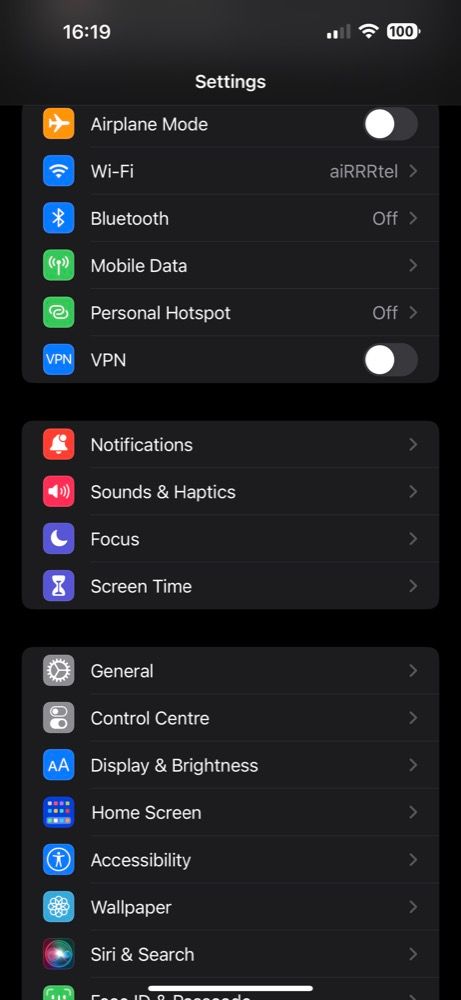This image depicts a colored screenshot of a person's iPhone settings screen. At the top, the time is displayed as 16:19. In the upper right corner, the phone shows two bars of cellular signal, full Wi-Fi coverage, and 100% battery life. The screenshot captures the Settings menu, listing various options including:

- **Airplane Mode:** A slider button that is currently off.
- **Wi-Fi:** Indicated by the label "AI-RRTEL."
- **Bluetooth:** Set to off.
- **Mobile Data**
- **Personal Hotspot**
- **VPN:** A slider button set to off.
- **Notifications**
- **Sounds and Haptics**
- **Focus**
- **Screen Time**
- **General**
- **Control Center**
- **Display and Brightness**
- **Home Screen**
- **Accessibility**
- **Wallpaper**
- **Siri and Search**

The descriptive text at the bottom of the screen is partially cut off and unreadable. The image is vertically oriented and contains no people, animals, plants, trees, or motorized vehicles.